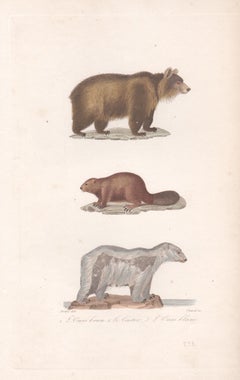This detailed image depicts a vertical drawing set against an ivory, yellowed, older book page background. At the top of the image, there's a large brown bear characterized by a thick mane of hair around its head, and a gradient of brown fur on various parts of its body. The bear stands on an oval patch of gray. In the middle of the image, there's a smaller brown beaver, distinctly featuring a long, slightly grayish tail and displaying an inquisitive posture, facing left while standing on a beaver-shaped gray oval. Finally, at the bottom, there's an animal that appears to be a polar bear, its primarily dirty white fur highlighted with darker gray shades along its body, standing on a rocky, light brown surface. Shadows are cast underneath each animal, adding depth to the illustration, and at the very bottom of the paper, there's a small saying in light gray text, which is too small to discern.